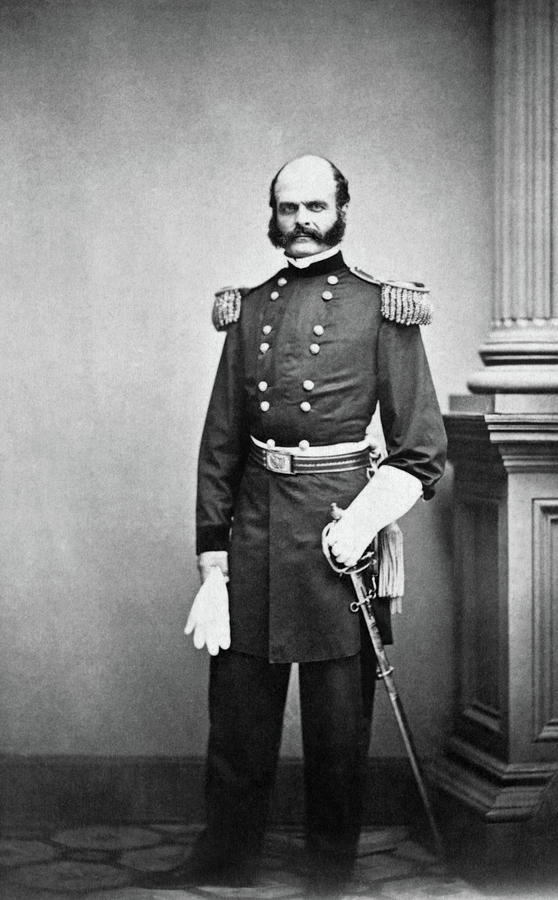This is a black and white photograph, estimated to be from the mid-1800s, possibly from the Civil War era. The image captures a man in a distinguished military uniform, suggesting he might be of high rank, potentially a general. He stands with a solemn expression, his receding hairline giving way to black hair on the sides of his head, which connect to prominent mutton chop sideburns and a notable mustache. His attire features a black, double-breasted coat adorned with gold-colored buttons, two sets of pairs on each side, and elaborate shoulder pads with hanging tassels. A sash and belt, characterized by black and silver lines, cinch his waist. 

In his right hand, he holds a white glove grasping a silver sword that reaches the floor, while his left hand holds another pair of white gloves. He stands on a black carpet patterned with gray circles, near a column that extends from the ceiling to a square base. The backdrop behind him is light gray, with a transition to darker gray at the top and bottom, complemented by a dark gray trim just above the floor. The photograph seems to have been taken in a studio, lending a formal and composed air to the scene.